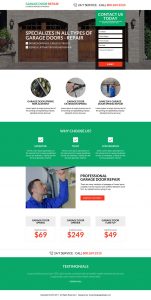This image presents a screenshot of a shopping website viewed on a cell phone. The overall quality is blurry, making detailed identification challenging. Dominating the lower portion is a prominent green bar with white text, its content indiscernible due to the blur. Just above this bar are three selectable options, each displaying a different price in red ink: $69, $249, and $49. Further up, there's a picture featuring a man wearing blue overalls and holding an unspecified object, with accompanying black text that is unfortunately illegible. Another green band with white text and selectable options sits at the very top of the image, though the specifics remain unclear due to the overall blurriness of the screenshot.